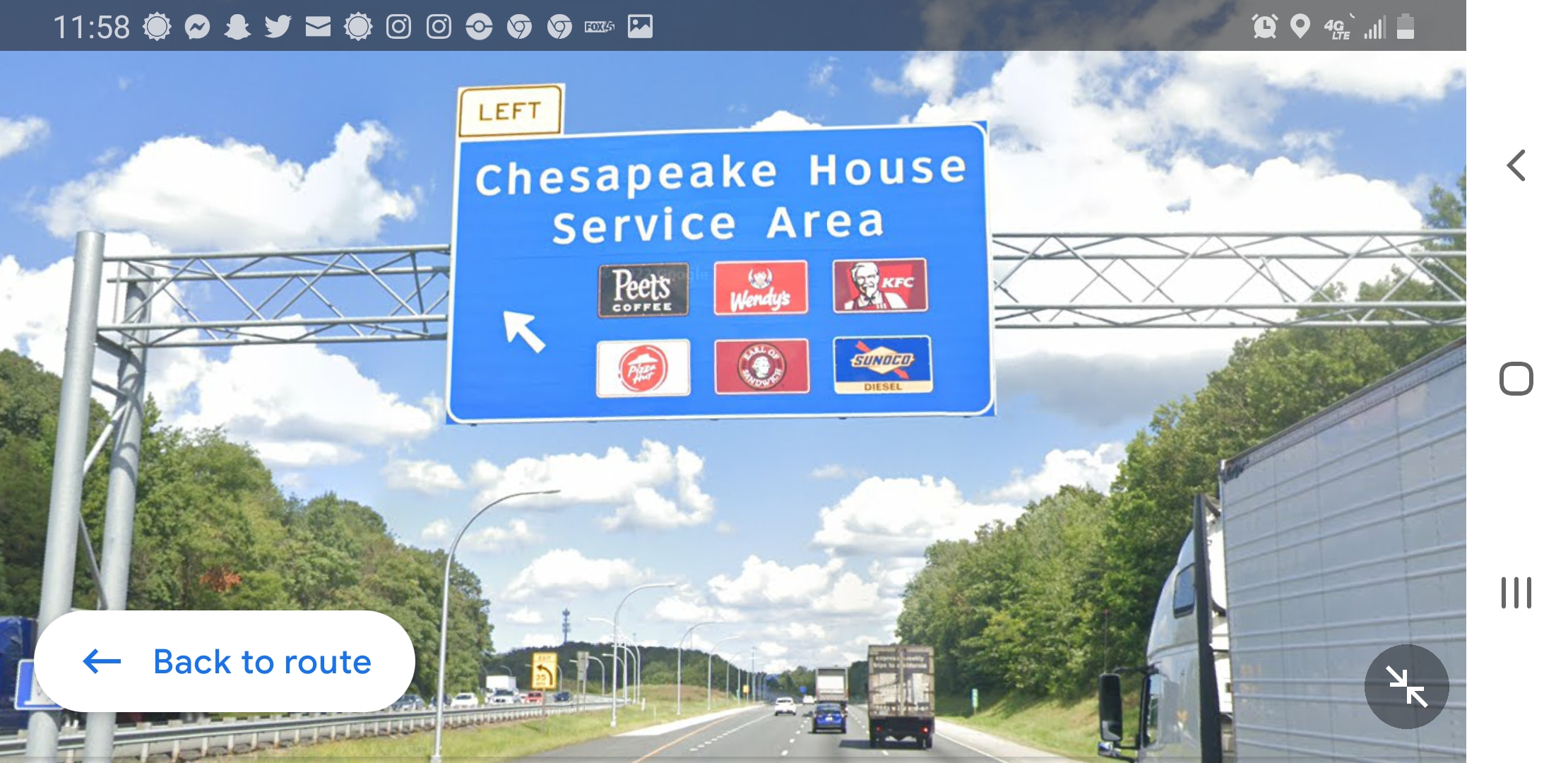This image is a screenshot taken from within a vehicle, depicting a highway scene. The landscape mode screenshot displays a bright blue sky adorned with thick, white, puffy clouds. At the top of the image, the time reads 11:58, along with several other icons typically found on a phone or computer screen. The road scene below is akin to a street view as if the viewer is driving down the road. On both sides of the highway, trees and grassy areas line the road, with a grassy median in the center.

In the background, a large, silver semi-truck is visible directly ahead, while several other tractor-trailers are seen traveling both ways. Spanning across the road is a large metal bridge or gantry, holding a blue sign with white text and trim. This sign reads "Chesapeake House Service Area," with a smaller accompanying sign at the top that says "Left" in black text. The sign includes logos for various eateries such as Pete's Coffee, Wendy's, KFC, Pizza Hut, and one presumed to be Panda Express. There is also a red circle sign and a gas station logo likely representing Conoco.

In the bottom left corner of the image, there's a white oval box with blue text that reads "Back to Route," alongside a left-pointing arrow. The bottom right corner contains another smaller icon, possibly a minimize button.